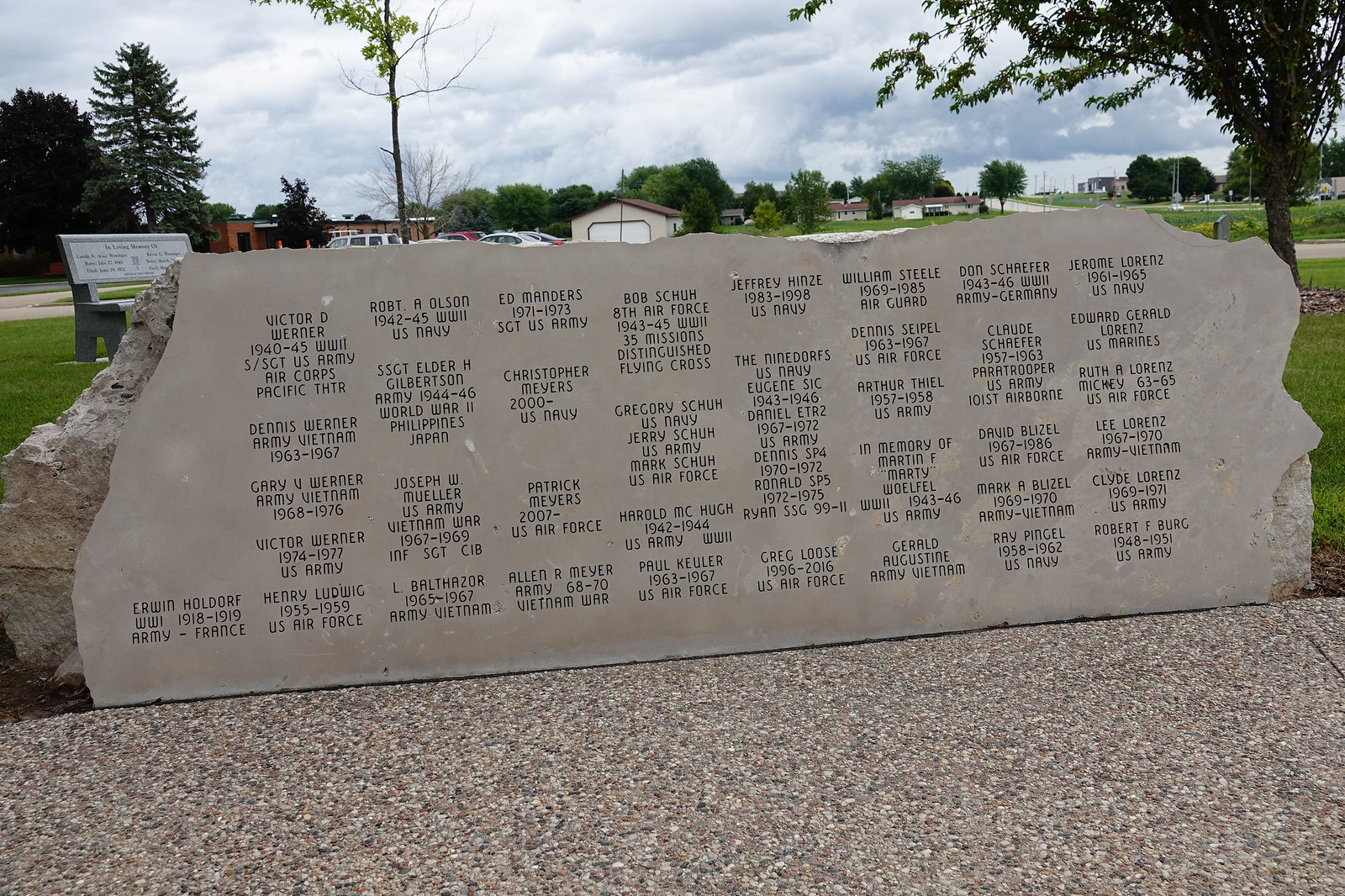The image features a gray, polished slate or granite monument, approximately five feet tall, prominently displaying the engraved names of around 35 to 40 individuals who have served and died in various wars. The names span multiple conflicts including World War I, World War II, the Vietnam War, and others; with details such as rank, service branches (Army, Navy, Marines, Air Force), and years of service (e.g., Erwin Huldorff, World War I, 1918-1919, Army, France; Victor D. Warner, 1940-1945, World War I, Staff Sergeant, U.S. Army, Air Corps, Pacific Theater; Gary V. Warner, Vietnam, 1968-1976, U.S. Army). This memorial is situated in a well-maintained park, evidenced by the surrounding grass, gravel walkway, and scattered trees. A stone bench in the background, inscribed with "In loving memory of...," suggests a somber dedication. The park environment includes visible elements such as a parking lot with cars, a shed, and the rooftops of nearby homes and buildings. This poignant setting serves as a tribute to the local community's military heroes.